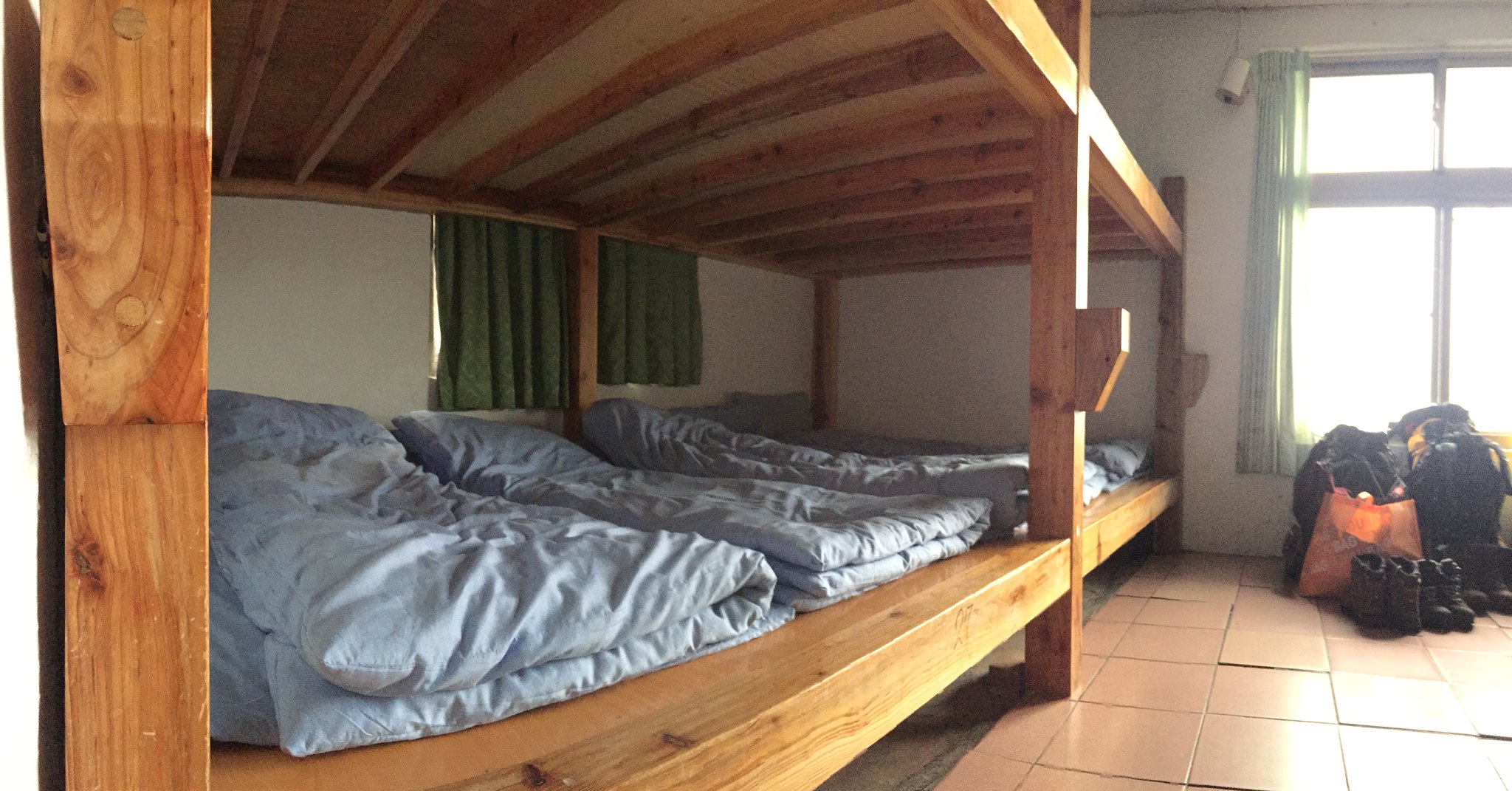The photograph depicts an indoor sleeping area, possibly in a hostel or a home. Dominating the left side of the image is a large, wooden bunk bed structure that angles from the foreground towards the center right. The bottom bunk features three neatly folded blue comforters. Behind the bunk bed on the back wall is a small window adorned with gray curtains. To the upper right, a large window with greenish-blue curtains pulled open allows bright sunlight to filter through, casting highlights on the bunk bed's wooden frame. On the floor in front of this window are signs of recent activity, with luggage, including several backpacks, and two pairs of black boots strewn about. The floor beneath is light-colored tile, some pieces of which are noticeably popped off. The overall ambiance suggests casual accommodation, perhaps a hostel, enhanced by the white walls and the mix of natural and artificial lighting.